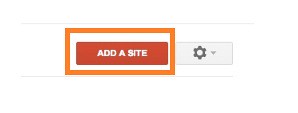This vertical screenshot, although small and heavily cropped, reveals an interface likely related to website creation instructions. Dominating the image is a large, thick, orange rectangle highlighting a red button with white text reading "Add a Site." The leftmost quadrant of the image is blank, filled with empty white space. Towards the right, a dark gray to black cogwheel icon, accompanied by a tiny upside-down triangle, suggests a drop-down menu where additional settings can be accessed or modified. Based on these elements, this screenshot appears to be a segment of a tutorial or guide for creating or adding a new website.